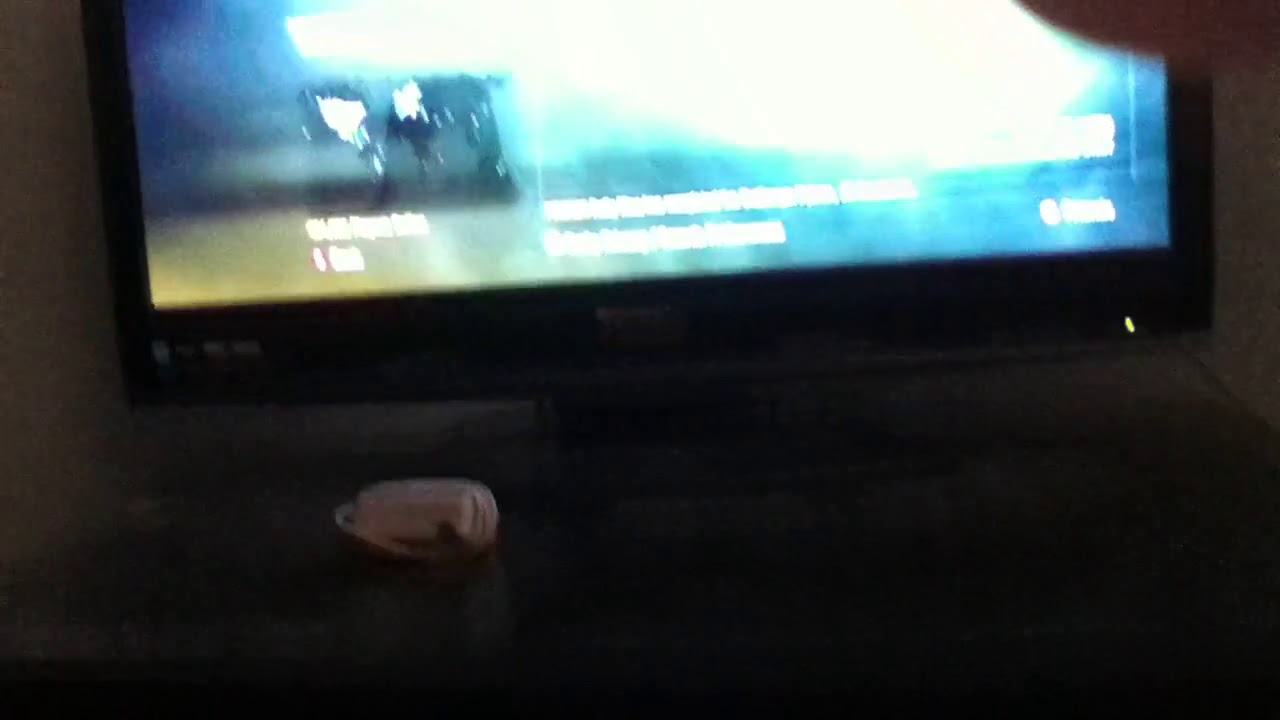This image, taken indoors and slightly blurred, depicts a rectangular-shaped photograph where the length exceeds the width. At the center is a display screen with a black boundary, emitting a blue-themed light interspersed with white text. The screen appears to be very bright, perhaps indicating it is a TV. The photograph is taken in a dark setting, further complicating visibility. In front of the TV screen, there is a distinguishable pink object. Additionally, there is a notable green light at the bottom of the TV, suggesting it is powered on. The TV seems to be placed on a stand, with a white, round-shaped plastic object—potentially a video game remote—positioned in front of it. Overall, the image is characterized by its lack of clarity and indistinct elements due to poor quality and blurriness.